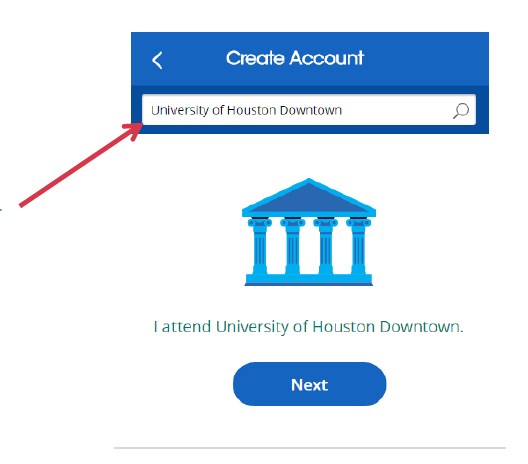This is a cropped screenshot of an app's "Create Account" section. At the top, a blue navigation bar bears the title "Create Account" in large white font, centered. To the left of the title is a white arrow pointing left. Just below the navigation bar, there is a substantial search bar with "University of Houston Downtown" typed into it. Adjacent to the search bar, in the bottom-left corner, a red arrow points diagonally towards the text inside the search box. The central portion of the screen features an image depicting a roof supported by pillars. Below the image, large gray text states, "I attend the University of Houston Downtown." Directly beneath this statement is a prominent blue button labeled "Next" in medium white font. At the very bottom of the screenshot, there is a gray horizontal line indicating where the image was cropped.